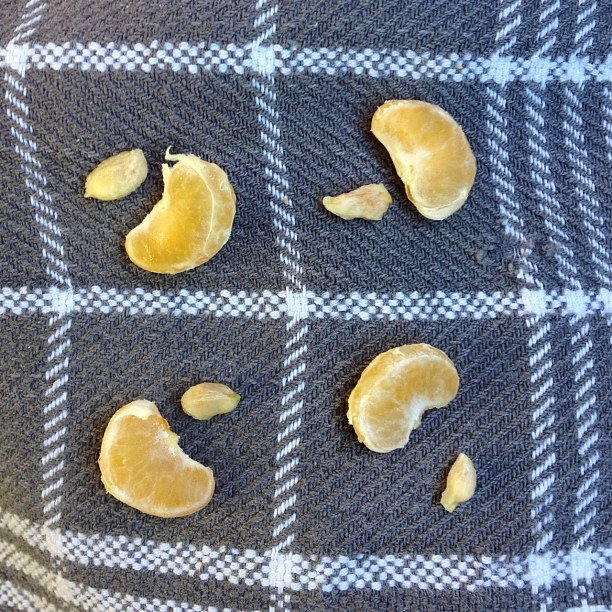This close-up photograph features four squares of a dark gray and light blue plaid fabric, possibly a dish towel, with a pattern of white checkerboard striping. On this fabric lie various slices of a small orange, which appear more yellowish than typical orange, suggesting they might be tangerine slices. Each square hosts a pairing of a larger and a smaller orange slice, accompanied by seeds. The towel is not completely flat, displaying some zigzagged lines due to curvature on the bottom left corner. The meticulous arrangement and intricate textile pattern give the image a detailed, almost artistic quality.